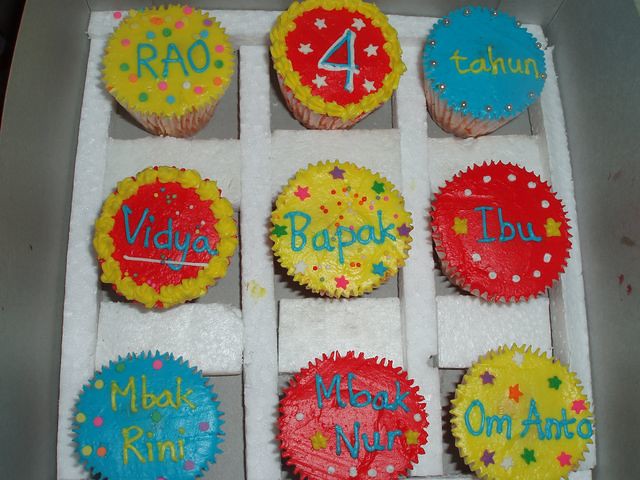This is a detailed photograph of nine homemade cupcakes arranged in a white styrofoam tray that forms a 3x3 grid. Each cupcake is nestled in its own compartment to prevent them from knocking into each other. The cupcakes are decorated with different colors of icing: three yellow, four red, and two blue. Each cupcake features colorful decorations like star-shaped sprinkles, dots, and silver beads, except one which prominently displays the number four. The cupcakes are personalized with various names and words spelled out in letters: "RAO" on a yellow cupcake, "4" with six white stars on a red cupcake, "TAHUN" on a blue cupcake, "BIDYA" on a red cupcake, "BACK" on a yellow cupcake, "IBU" on a red cupcake, "Mbak Rini" on a blue cupcake, "Mbak Noor" on a red cupcake, and "Omanto" on a yellow cupcake. The vibrant display and the presence of the number four suggest that this arrangement might be for a birthday celebration.